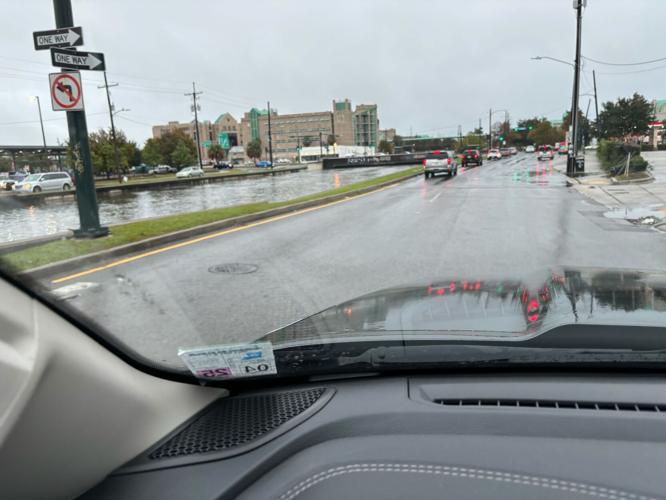In this photo taken from the driver's seat of a black SUV or truck during a rainstorm, the viewer is given a perspective through the front windshield on a dreary, wet day in what appears to be a town or city. The rain has dampened the road and left droplets on the windshield. In the lower left corner of the window, a registration and possibly an inspection sticker are visible. Ahead, multiple vehicles are seen idling in traffic. Street signs to the left indicate a one-way road and a no-left-turn rule, while telephone poles, power lines, and a mix of trees and buildings add to the urban landscape. The scene is accented with various colors including red, teal, tan, black, gray, white, and green, with the green on a tan building standing out prominently amidst the overcast conditions.